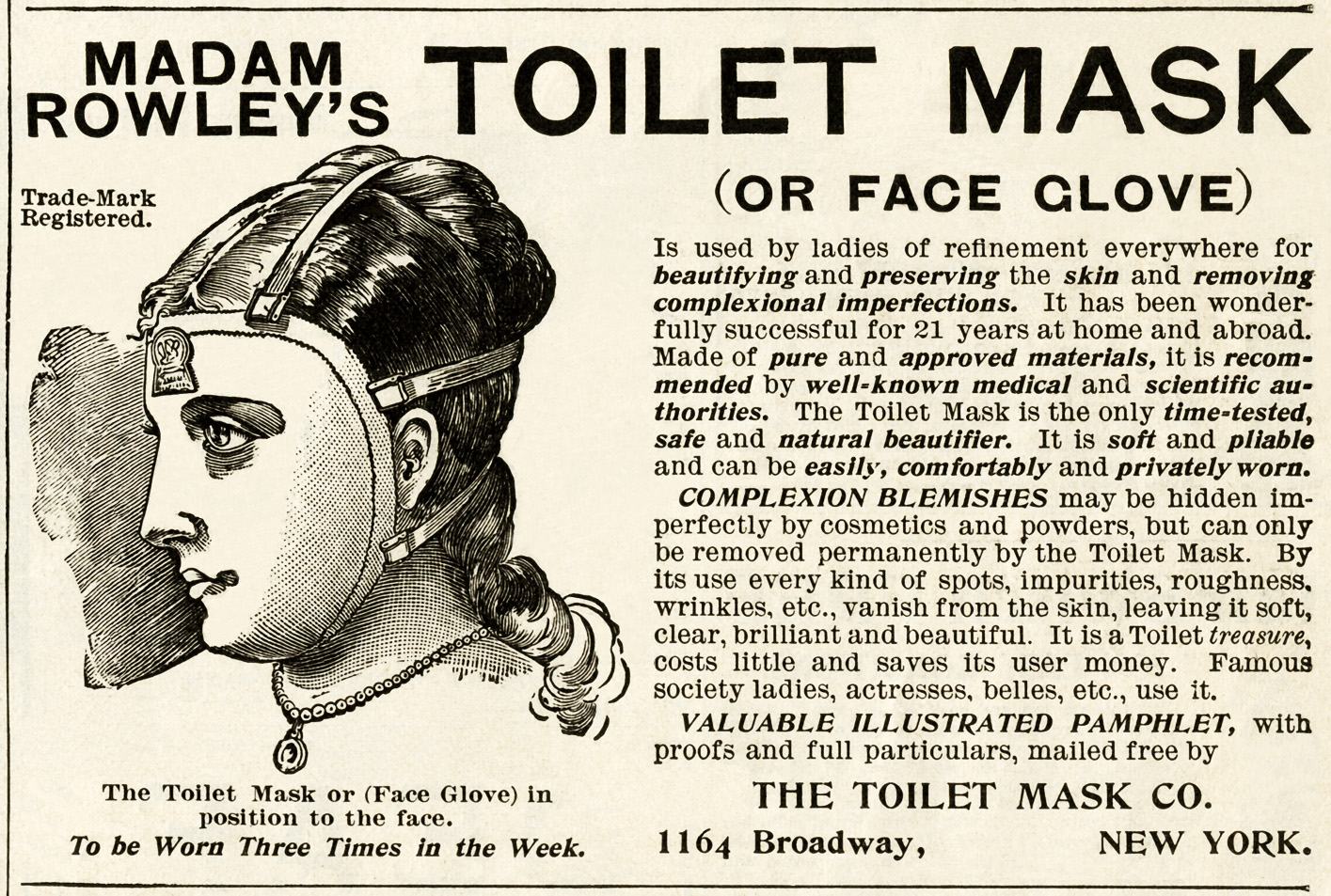This image is a vintage newspaper advertisement for Madam Rowley's Toilet Mask, also known as the Face Glove. The ad features a black ink illustration on yellowish paper, showing a woman with dark, braided hair and a pearl necklace, wearing the white mask held by bands. The mask is described as a time-tested, natural, and safe beautifier used by society ladies, actresses, and belles for 21 years at home and abroad. It is made of pure, improved materials recommended by medical and scientific authorities. The Toilet Mask is to be worn three times a week to beautify and preserve the skin, permanently removing blemishes, spots, impurities, roughness, and wrinkles, leaving the skin soft, clear, and radiant. A valuable illustrated pamphlet with proofs and full details is available for free by the Toilet Mask Company at 1164 Broadway, New York.